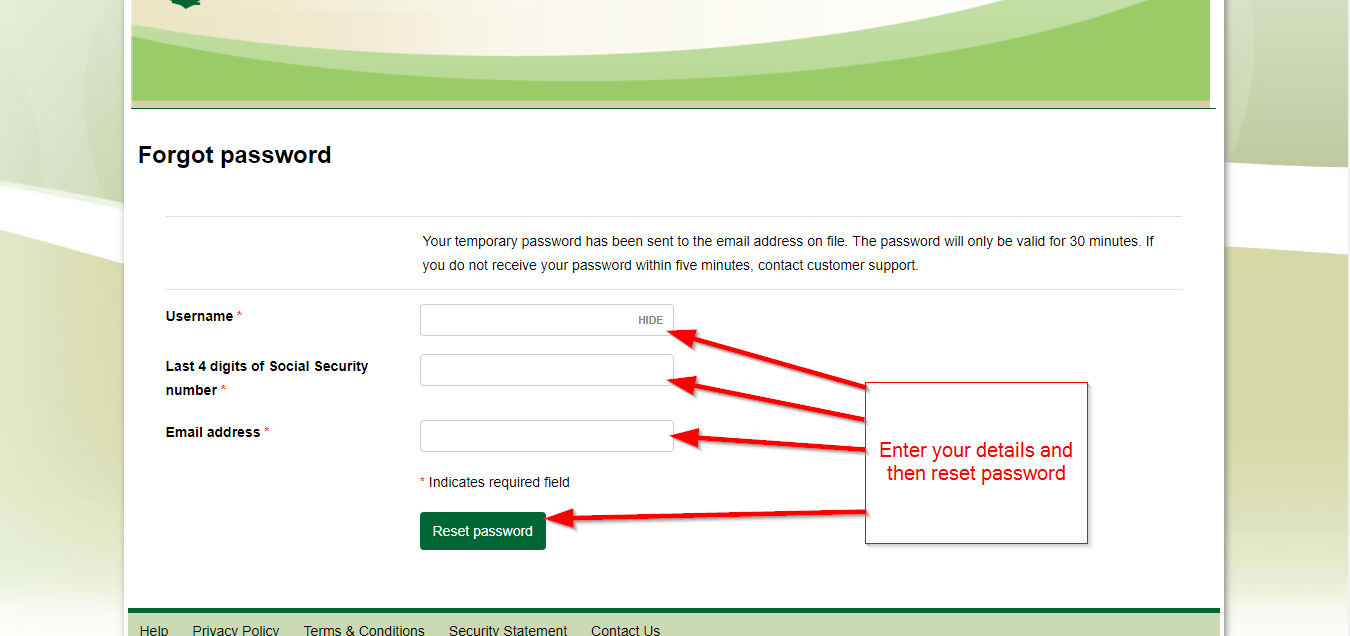The image captures a computer screen with a predominantly gray background. Near the top center, a white, curved line runs horizontally across the gray backdrop. Positioned centrally on the screen, covering most of the background, is a pop-up window featuring a colorful design at the top with shades of pink, light green, and dark green. 

Below this decorative header, the pop-up window has a white background that contains text and form fields. The text reads: "Forget Password." Further instructions in small print detail that a temporary password has been sent to the email address on file, specifying that the password will be valid for 30 minutes. Additionally, it suggests contacting customer support if the password is not received within five minutes.

Beneath these instructions, the user is prompted to enter their username, last six digits of their social security number, and email address. The form fields for these inputs are aligned vertically, with a note indicating that these fields are required. 

At the bottom of the form, a prominent green button labeled "Reset Password" invites the user to proceed. Enhancing clarity, a red arrow directs attention from the form fields to a square on the side, containing the text, "Enter your details and then reset password," providing a step-by-step guide for the process.